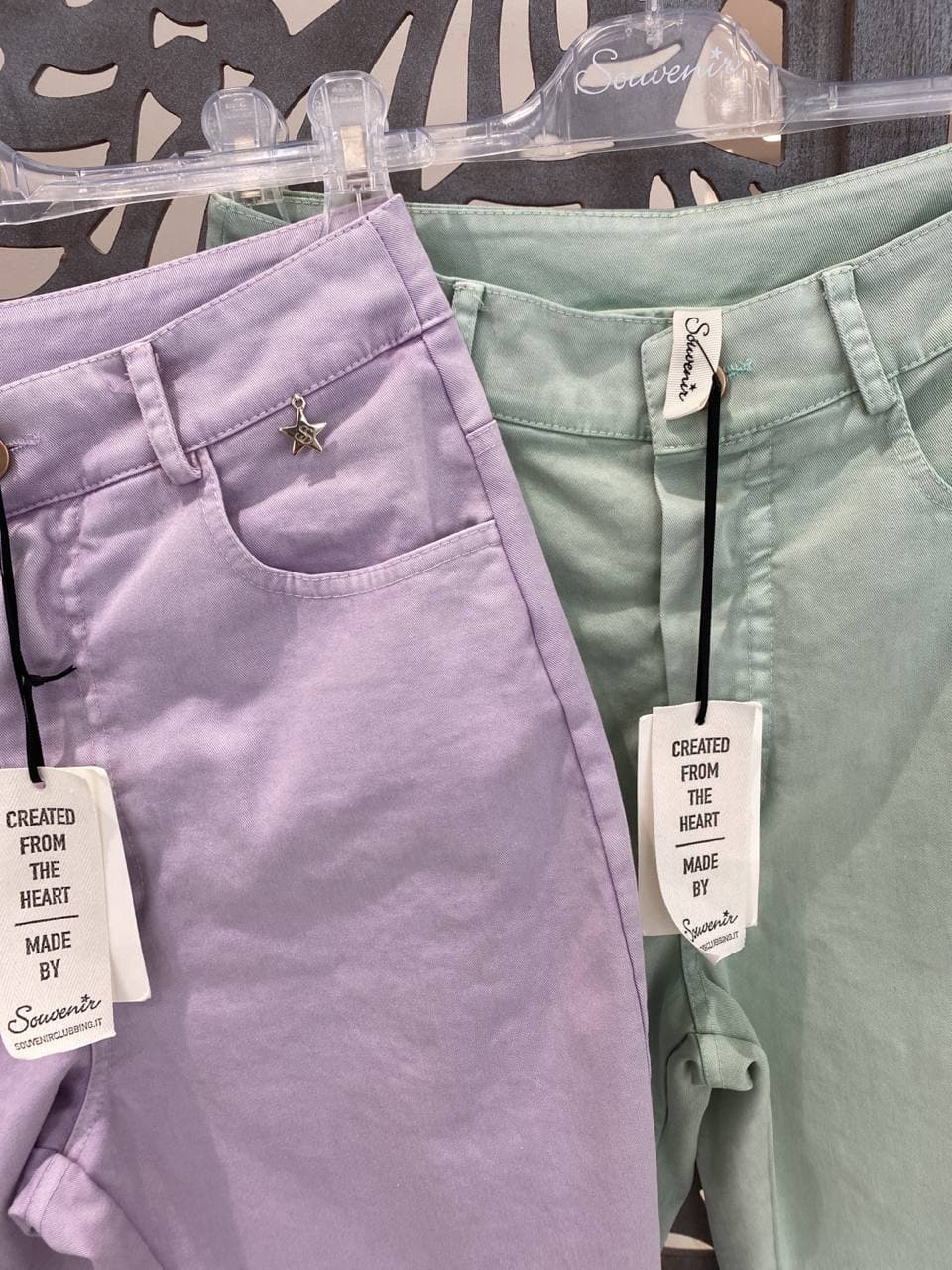The photograph showcases two pairs of pastel-colored denim jeans hanging on clear hangers against a wall featuring black and white wavy, stencil-style cutouts. The pair on the left is light purple, adorned with a small silver star charm hanging near the front left pocket, attached by a loop to the waistband. The charm appears to have interlocking "SS" initials engraved on it. Both pairs of jeans have informational tags hanging from black strings attached to the buttons at the waist. The tags read "Created from the heart, made by Souvenir," with "Souvenir" written in cursive. The pair on the right is a pastel lime green color, and while partially obscured by the purple jeans, the tags and attachments are similarly styled. The close-up shot primarily captures the upper sections of both pairs of jeans, emphasizing their intricate details and delicate, spring-like hues.